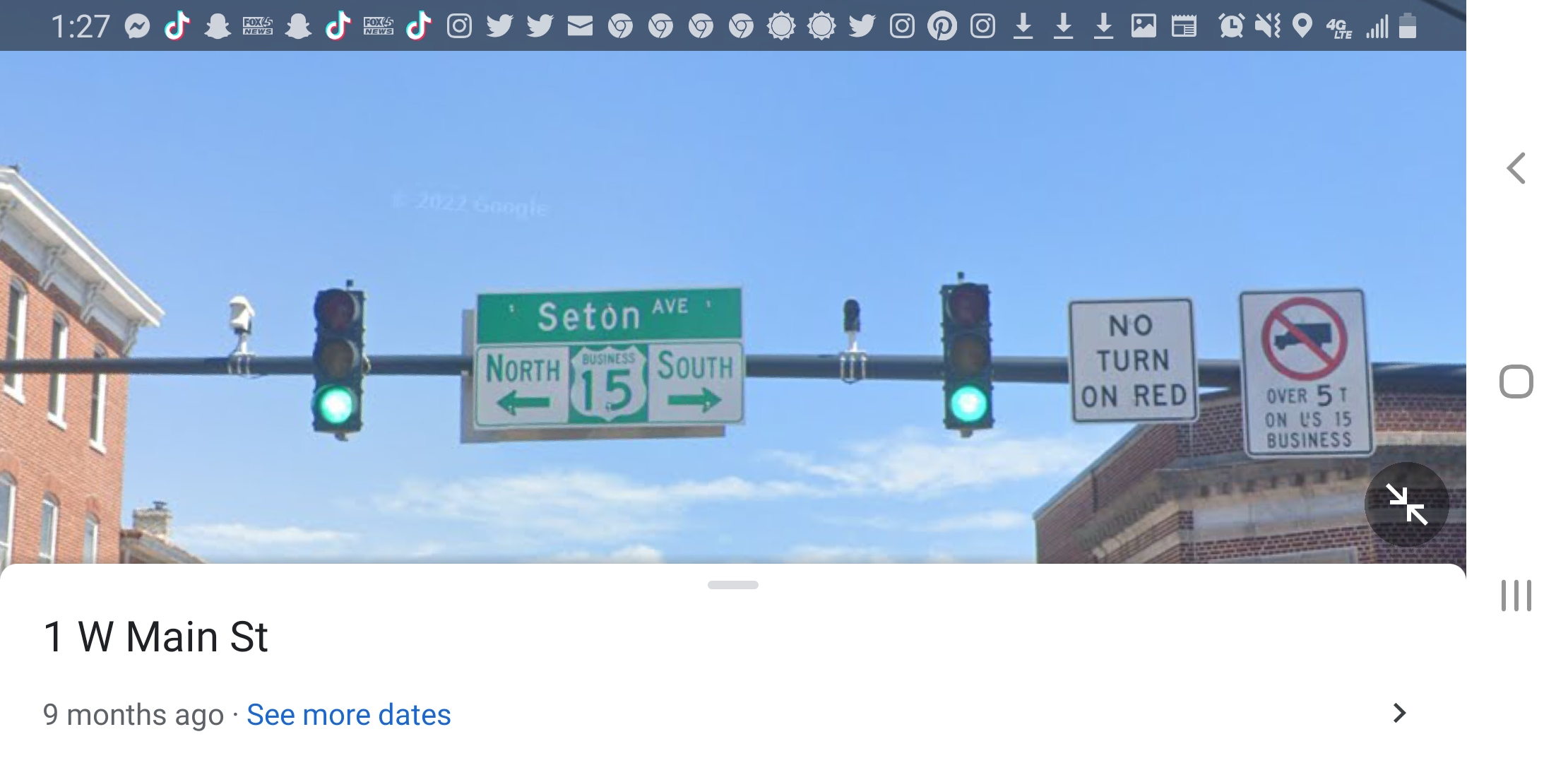An image captured from a phone or tablet, likely from a website, displays a horizontally rectangular scene dominated by traffic lights and street signs. At the top of the image, a thin gray banner indicates the time as 1:27, flanked by numerous app icons, including Messenger, Snapchat, Twitter, and TikTok, among others, as well as icons for an alarm, speaker, location, signal strength, and battery status. Below this bar, the image showcases a clear blue sky framed by buildings on the left and right. Stretching horizontally across the scene is a long metal bar supporting traffic lights. Starting from the left, a green traffic light is followed by a rectangular green sign labeled "Seton Avenue," pointing left for north and right for south, with a business route 15 designation. Adjacent to this is another green light, a "No Turn on Red" square sign, and a "No Trucks Over 5 Tons" rectangular sign. The composition centers on the intersection, providing a detailed snapshot of urban street signage under a clear sky.